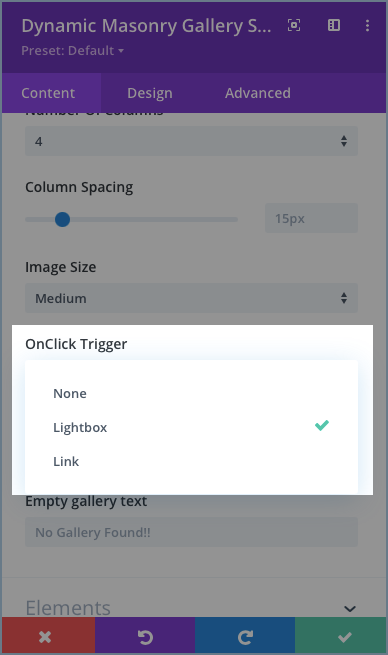This is a detailed screenshot of a mobile phone's interface, depicting the settings menu of a "Dynamic Masonry Gallery". The background of the screen is dimmed, highlighting an active white dialog box in the forefront. The dialog box is titled "On Click Triggering" and presents a list of options: "None," "Lightbox," and "Link," with "Lightbox" selected and marked with a blue checkmark.

At the top of the screen, there is a blue strip that transitions into a purple strip below. The blue strip contains the title "Dynamic Masonry Gallery" and a "Preset Default" label. Below the purple strip, there are three tabs labeled "Content," "Design," and "Advanced," arranged horizontally from left to right.

The main content area of the page is white, featuring a grey strip that spans the width of the screen. This grey strip includes the number "4" and the label "Column Spacing" with a sliding control to adjust the spacing. Below this is a label "Image Size," and underneath, there is an empty white box marked as "Gallery Text Elements."

At the bottom of the screen, there is a series of buttons spanning the width of the interface with distinct colors: a red button with an "X" symbol, a purple button for rewinding to the left, a blue button for rewinding to the right, and a green button with a checkmark.